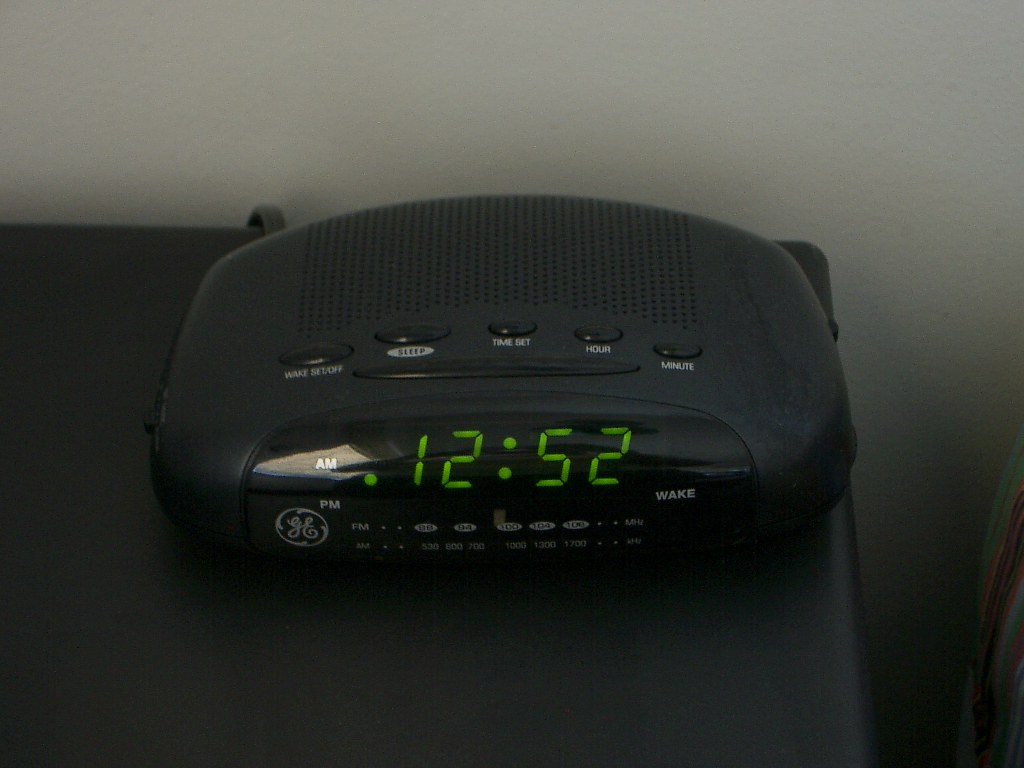The photograph showcases a black, pillow-shaped General Electric clock radio resting on what appears to be a black nightstand. The clock features a lime green digital display indicating the time as 12:52, with an AM and PM indicator where the green dot is positioned halfway between them, making it unclear whether it's AM or PM. The clock face includes a General Electric logo in the bottom left corner. Below the display, there is a dual radio dial with the FM band on top and the AM band beneath it. The clock radio is equipped with several function buttons along its curved top, including modes for wake, set or off, sleep, time, hour, and minute settings. The housing of the clock radio is black, and it has evenly spaced holes where the speaker is located. The text on the buttons is written in white ink, providing clear labels for each function.